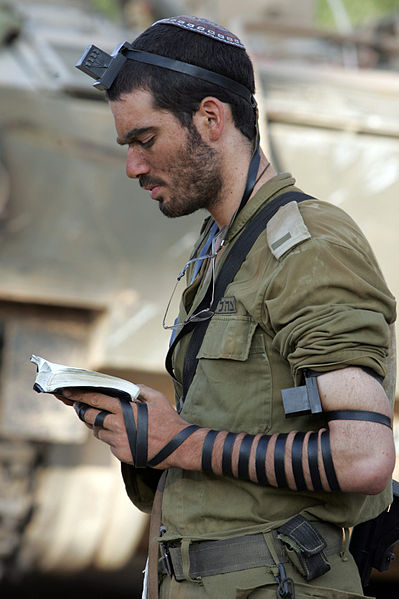In this full-color daytime photograph, an Israeli soldier, identifiable by his military fatigues, stands facing left. Sunlight glints off a metallic surface—likely a military vehicle—in the upper right corner, confirming the daylight setting. The soldier, a young male with short dark hair and a short black beard, wears a yarmulke and a small black protrusion on his forehead, possibly a religious object. He is deeply engrossed in reading a book, which could be the Torah, held in his hands. His military attire includes a long-sleeved shirt with the sleeves rolled up to his elbows and a belt at his waist, beyond which the image is cut off. Around his neck, he has a strap with glasses hanging down and another black and blue item. Notably, a black leather strap, known in Jewish tradition as tefillin, wraps intricately around his left arm: a single band starts above the elbow and wraps multiple times down the forearm, encircling his wrist, and continues between his thumb and forefinger with additional loops around his middle finger.